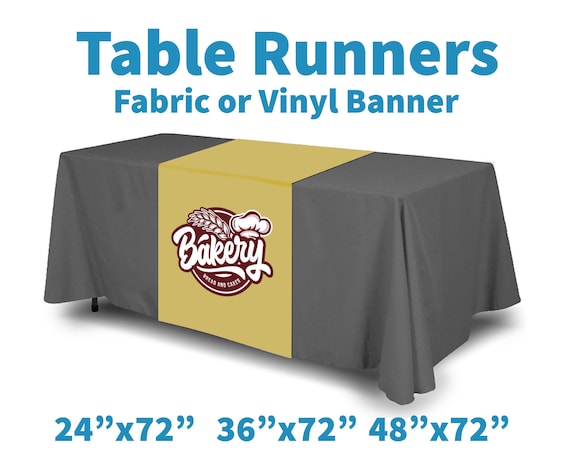This horizontal advertisement showcases custom table runners or banners, available in fabric or vinyl. At the center of the image is a long table draped in a dark gray tablecloth with a prominent beige stripe running through the middle. This stripe extends over the edge of the table. The front-facing section of the tablecloth features a bakery-themed logo within a brown symbol, displaying the word "Bakery" in elegant white lettering beside a graphic that includes a chef's hat and wheat. Positioned above the table in bold blue text are the words "Table Runners" and "Fabric or Vinyl Banner." The advertisement also lists available sizes for the table runners: 24" x 72", 36" x 72", and 48" x 72", catering to various table dimensions.